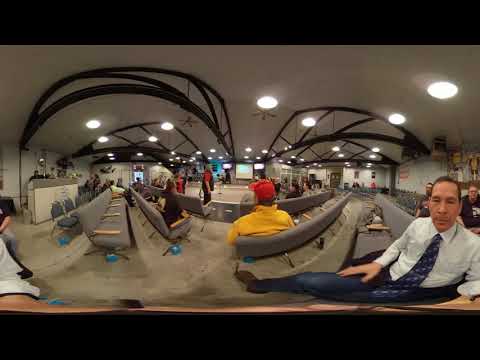This photograph captures a unique panoramic, fisheye view of an indoor space that appears to be a waiting area or office building. The image is split into two distinct fisheye views, one on the left and one on the right, providing a broad perspective of the room.

The room features a light gray floor and a white ceiling adorned with circular white lights, curved black metallic beams, and some fans. Two archways are visible within the space, adding architectural interest. The seating in the room is arranged in rows, reminiscent of theatrical style seating, facing towards the center of the room. These seats curve around a central area, which might be an open space or a big screen.

On the left side, beneath the archway, there are three rows of side-by-side seats, with a carpeted elevated area behind them, also lit by overhead white lights. On the right side of the image, a similar seating arrangement can be seen extending back into the background.

In the foreground on the right, a man dressed in a white button-down shirt, blue tie, and navy pants is taking a selfie, looking into the camera with his arm extended unnaturally due to the panoramic effect. His attire suggests he might be a businessman. Another man, closer to the center, is seen facing away from the camera, wearing a yellow-gold jacket and a red baseball cap. He appears to be looking toward the central open area or screen.

The room’s design and furnishings, including the seating and lighting, suggest it may be an area designed for waiting or leisure, possibly within a travel terminal or office building.